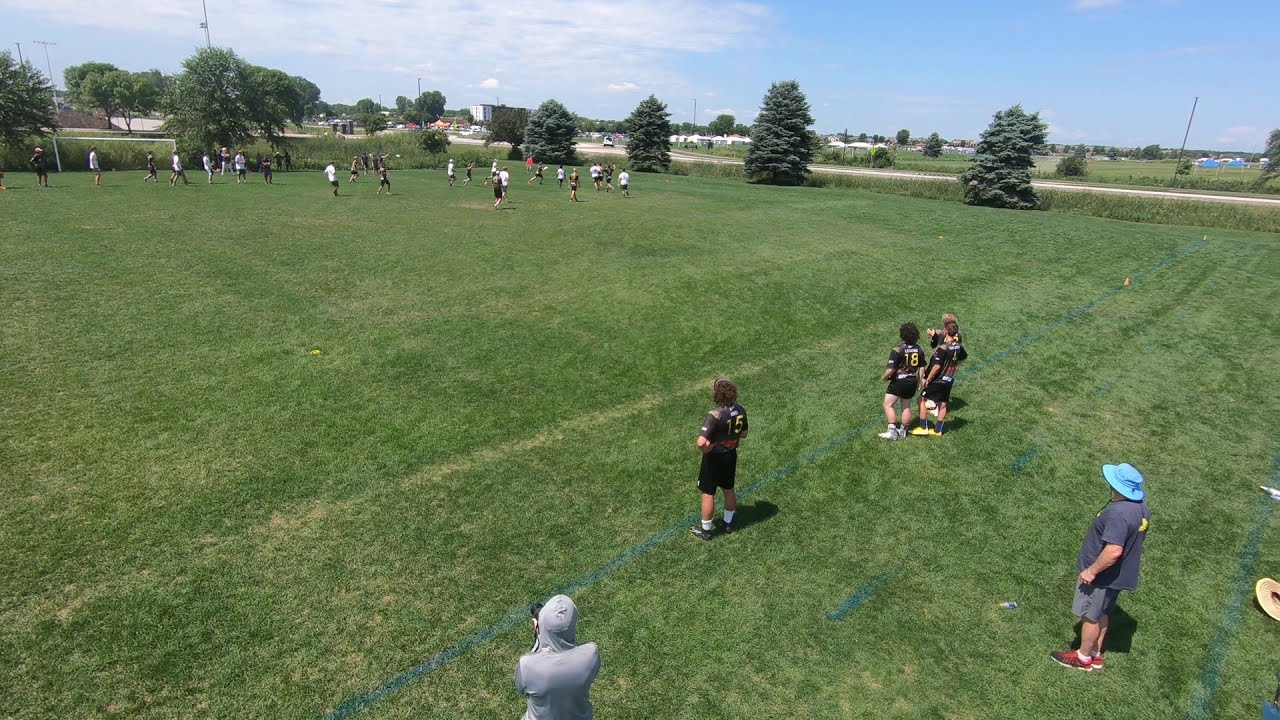The image captures an outdoor scene on a sunny day with light blue skies dotted with a few clouds. From a slightly elevated vantage point, approximately 15 feet off the ground, we are looking down at an expansive, well-kept grassy field, bordered in the distance by a rectangular line and a few trees. The predominant focus is on a soccer match in progress, evidenced by the movement of players scattered across the green field. Players are dressed in contrasting uniforms— some in dark jerseys and shorts, others in light or white jerseys— though the exact team formations are not perfectly clear. The goal is visible in the top left section of the image.

In the foreground, close to the sidelines of the match, stand several onlookers. Among them are two adults: one wearing a light blue hat and a purplish t-shirt paired with gray pants, another in a gray hoodie, potentially taking photographs. Beside them are three or four older children or young adults in black jerseys and shorts, likely players waiting to substitute into the match. The entire scene is enveloped by the vibrant greenery of the field, without apparent borders or edges, emphasizing the vastness of the space.